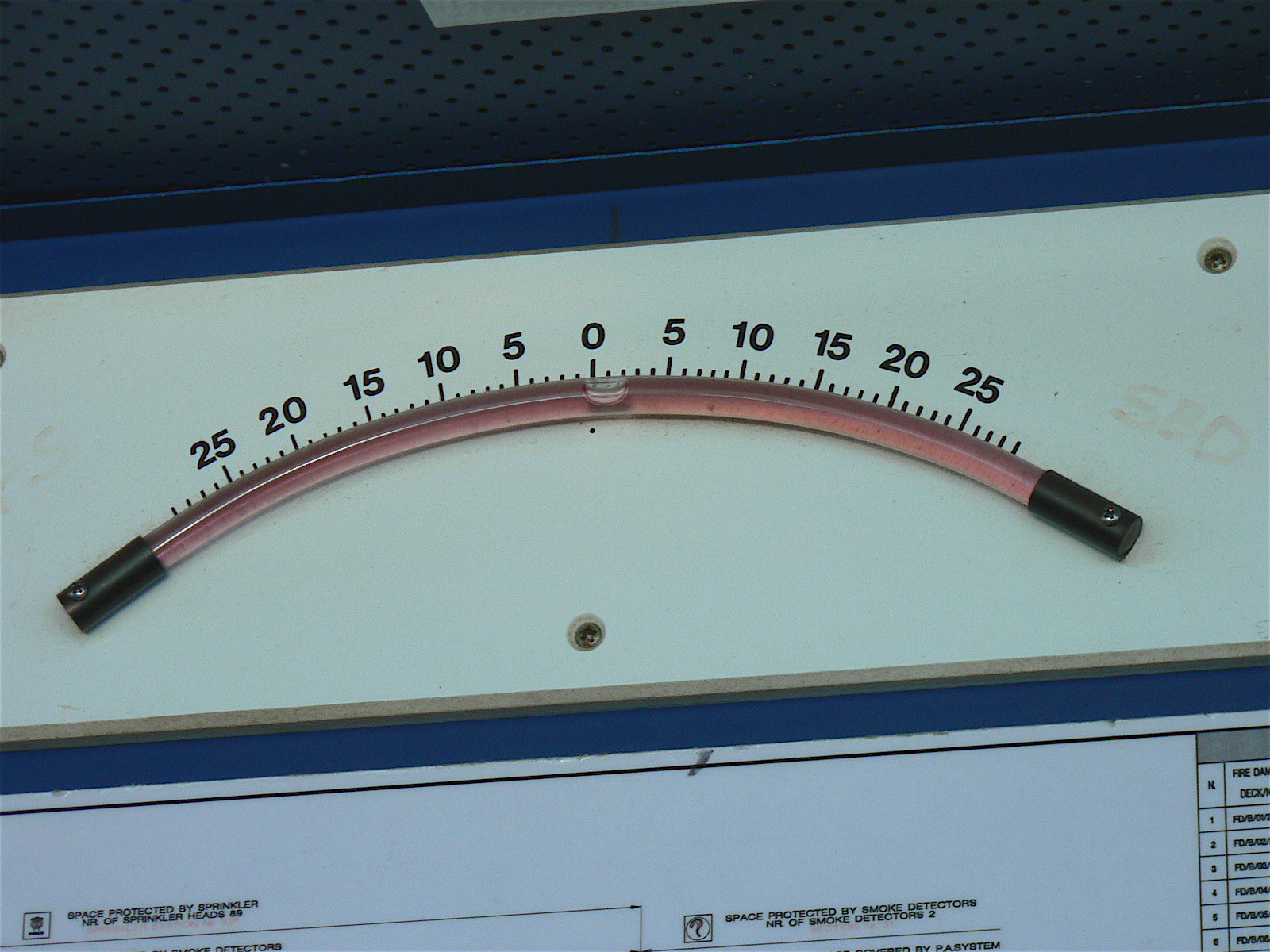The image showcases a close-up view of a monitoring device. At the top of the image is a dark navy-blue section. Below this, centrally positioned, is the main dial of the monitor. The dial features a white background bordered by a dark blue frame and presents an arched display. The display spans from black on either end to red in the center, forming a rainbow-like shape. The scale is marked with increments: 25, 20, 15, 10, 5, and 0 in the center, then ascending 5, 10, 15, 20, 25 to the right.

Below the dial is a white section with small black text, partially cut off. On the left, it reads: "Space protected by sprinkler, NR of sprinkler heads: 89." On the right, it states: "Space protected by smoke detectors, NR of smoke detectors: 2." In the bottom left corner, there's additional writing and numbers, but most of it is obscured, displaying only: "1, 2, 3, 4, 5, 6."